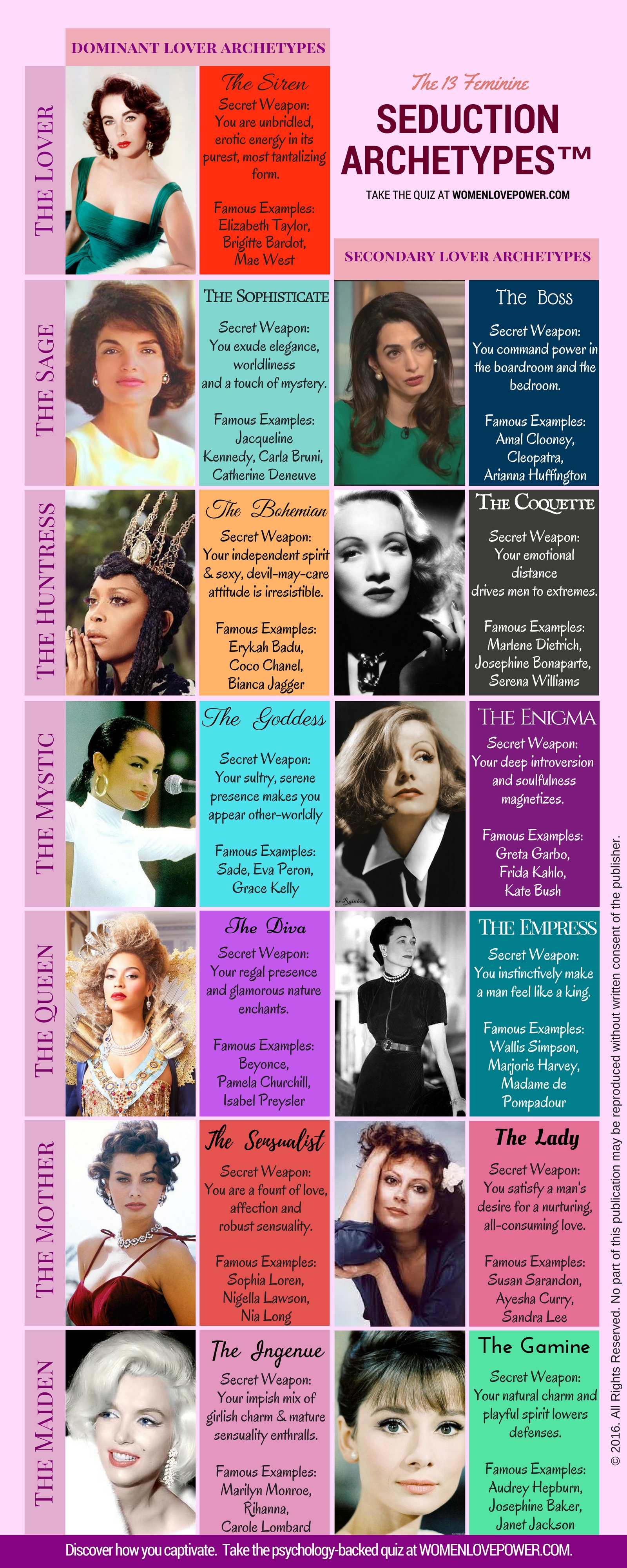The image titled "This is Feminism, Seduction Archetypes" is a detailed graphic with a pink background that categorizes various feminine archetypes into dominant and secondary lover archetypes. At the top, the graphic invites viewers to "take the quiz." 

On the left side, it lists dominant lover archetypes including categories such as the Lover (represented solely by the Siren), the Sage (the Sophisticate), the Huntress, the Mystic, the Queen (the Diva), the Mother, and the Maiden. On the right side, it highlights the corresponding secondary lover archetypes, such as the Boss (under the Sage), the Empress (under the Queen), among others.

Each row features one dominant and one secondary archetype, which are distinctly colored in shades like red, yellow, blue, purple, green, and pink for easy differentiation. Adjacent to each archetype's description is a photo of a famous woman or character that exemplifies that archetype. The images serve as visual representations of each category, making the comparisons and attributes clear.

At the bottom of the image, there's a purple bar with white text for additional information or instructions. Overall, the image is an intricate, color-coded chart that visually encapsulates the variety of feminine seduction archetypes.